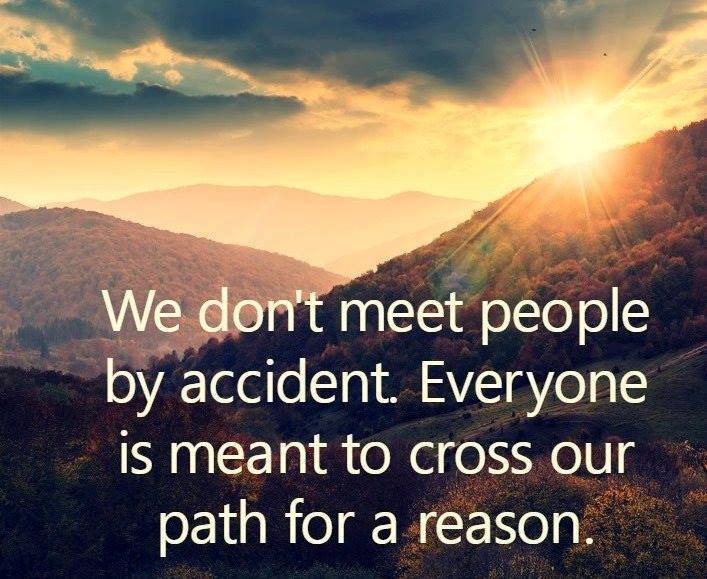The image captures a serene, mountainous landscape in autumn, with nearby hills adorned in a vibrant tapestry of orange, red, and yellow foliage, accented with touches of green. The scene is bathed in the warm, golden hues of a setting sun peeking over the right-hand side of the hills, casting an enchanting glow that illuminates the sky with shades of orange, yellow, and pink. Dark clouds hang dramatically above, contrasting against a hint of blue sky in the upper left corner. In the distance, mist-covered peaks appear as orange silhouettes on the horizon. The image, rectangular and poster-like in shape, measures approximately six inches wide by five inches tall. At the bottom, a poignant quote in bold, white text reads, "We don't meet people by accident. Everyone is meant to cross our path for a reason," overlaying the tranquil and picturesque background.